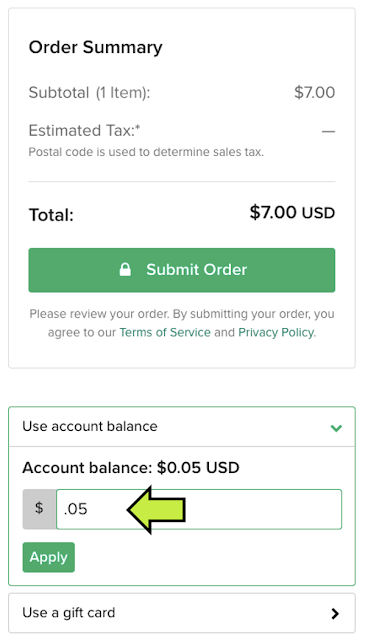A detailed caption for the screenshot could be:

"Screenshot of a web page displaying an order summary for an online purchase. At the top, the heading 'Order Summary' is prominently displayed in bold. The summary lists the subtotal for one item priced at $7. Below, it mentions 'Estimated Tax' but indicates that the postal code is required to determine the sales tax, leaving this field blank with a placeholder line. The total cost is specified as $7 USD, highlighted in bold.

A green 'Submit Order' button with white text and a white lock icon is prominently featured, accompanied by the instruction 'Please review your order. By submitting your order, you agree to our Terms of Service and Privacy Policy,' with 'Terms of Service' and 'Privacy Policy' presented as clickable dark green links.

Towards the bottom, there is an option to 'Use Account Balance' with the account balance of $0.05 USD stated in bold text. An icon of a black arrow indicates that the user can apply this balance. Another option, 'Use a Gift Card,' is provided at the bottom with a corresponding arrow, both enclosed in green and gray boxes, respectively."